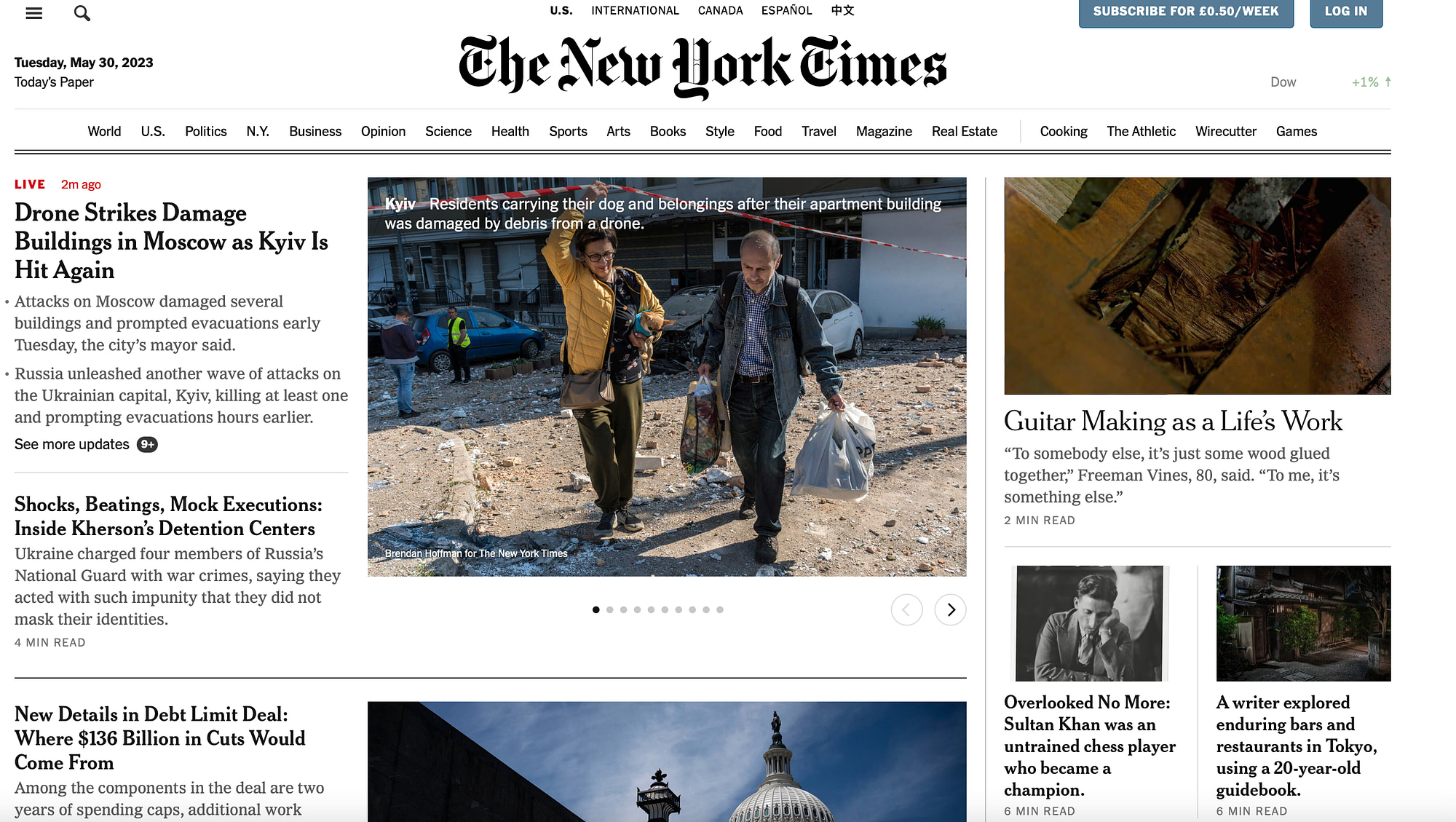**Front Page of The New York Times - Tuesday, May 30th, 2023**

**Main Headline:**  
- **Drone Strikes Cause Severe Damage in Moscow**  
  Attacks on Moscow early Tuesday resulted in significant damage to multiple buildings and triggered evacuations. The image shows a woman and a man, accompanied by their dog, carrying belongings out of their damaged apartment. Meanwhile, Russia conducted another wave of attacks on the Ukrainian capital, killing at least one person and prompting further evacuations.

**Additional Headlines:**  
- **War Crimes Charges Filed Against Russian National Guard**  
  Ukraine has charged four members of Russia's National Guard with war crimes, accusing them of engaging in torture practices including shocks, beatings, and mock executions within Kremlin detention centers. The individuals are reported to have acted with such impunity that they did not bother to conceal their identities.  

- **New Details on Debt Limit Deal**  
  New information reveals that the deal on the debt limit includes budget cuts amounting to $136 billion. The reductions will affect various sectors as the specifics of the agreement come to light.

- **The Art of Guitar Making**  
  For one individual, guitar making is more than the simple assembly of wood and glue; it is a lifelong passion and craft. The caption contrasts this deep appreciation with the perspective of others who may see it as merely a mechanical process.

- **Remembering Sultan Khan**  
  Sultan Khan, a previously overlooked, untrained chess player, rose to become a celebrated champion. His remarkable journey and contributions to chess are highlighted in this feature.

- **A Writer's Nostalgic Journey Through Tokyo**  
  In a nostalgic exploration, a writer delves into the enduring bars and restaurants of Tokyo using a guidebook that is two decades old, offering a glimpse into the city's rich and evolving cultural tapestry.

The front page captures a wide array of stories, reflecting both immediate global events and enduring human interests.